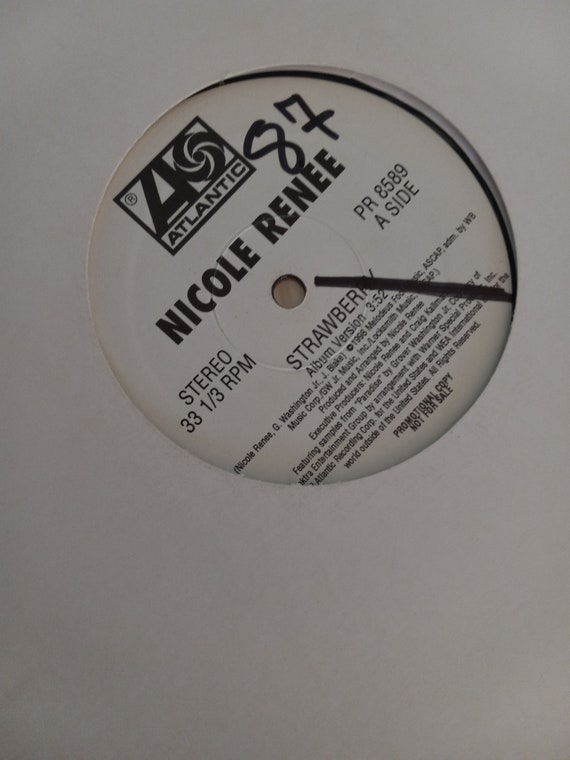This up-close photograph features the center label of a vinyl record encased in a white paper sleeve with a circular cutout, revealing essential details about the record. The label text showcases the artist, Nicole Renee, and indicates that the record is an Atlantic release (catalog number 87). The song featured is titled "Strawberry" (Album Version), with a playtime of 3:52 minutes. This is the A-side of the record, with the catalog number PR 8589. The record is a stereo format, playing at 33 1/3 RPM. Additional details such as information about the producers and the creation process are also present, although not fully visible in the image. At the bottom of the label, the text "Promotional Copy - Not for Sale" is prominently displayed, indicating that this vinyl is a promotional issue. The entire label text is rendered in black on a white background, characteristic of a typical vinyl record informational label.